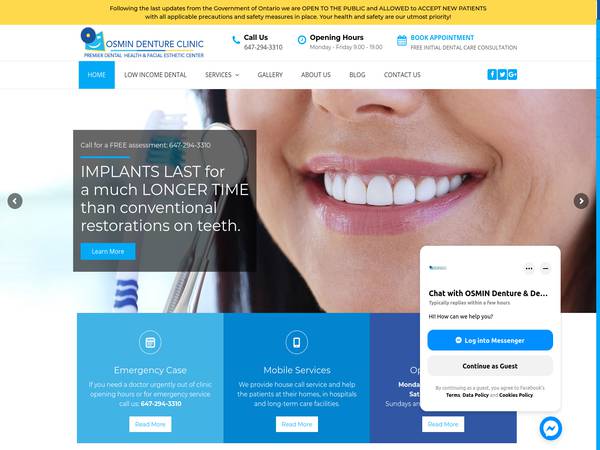This is an image of a screenshot from the Osmond Denture Clinic webpage. At the very top of the page, there is a thin yellow bar with a message stating: "Following the latest updates from the government of Ontario, we're open to the public and allowed to accept new patients with all applicable precautions and safety measures in place. Health and safety are our utmost priority."

In the top left corner, the clinic’s logo is displayed, featuring a graphic that resembles a bluish mountain-like shape with a darker blue circle to its left. The clinic's name, "Osmond Denture Clinic," is prominently featured to the right of the logo.

Below the logo, there is a navigation menu and contact information. The menu items include "Call Us," with the phone number (647-294-3310), and "Opening Hours," although the specific days and times are not visible. There is a "Book Appointment" button on the right side of the menu.

The main menu bar contains the following items: "Home" (highlighted in blue), "Low-Income Dental Services," "Gallery," "About Us," "Blog," and "Contact Us." 

The central part of the image features a smiling woman with straight white teeth, wearing pink lipstick. The background includes a grey box with white text stating, "Implants last for a much longer time than conventional restorations on teeth."

At the bottom of the image, three blue boxes are displayed in varying shades. The first box, in sky blue, says "Emergency Case" with additional text underneath. The second box, in a medium blue shade, indicates "Mobile Services." The third box is a royal blue color but its content is not described.

This detailed layout highlights the clinic's responsiveness to public health updates and emphasizes their dental services and patient care commitment.